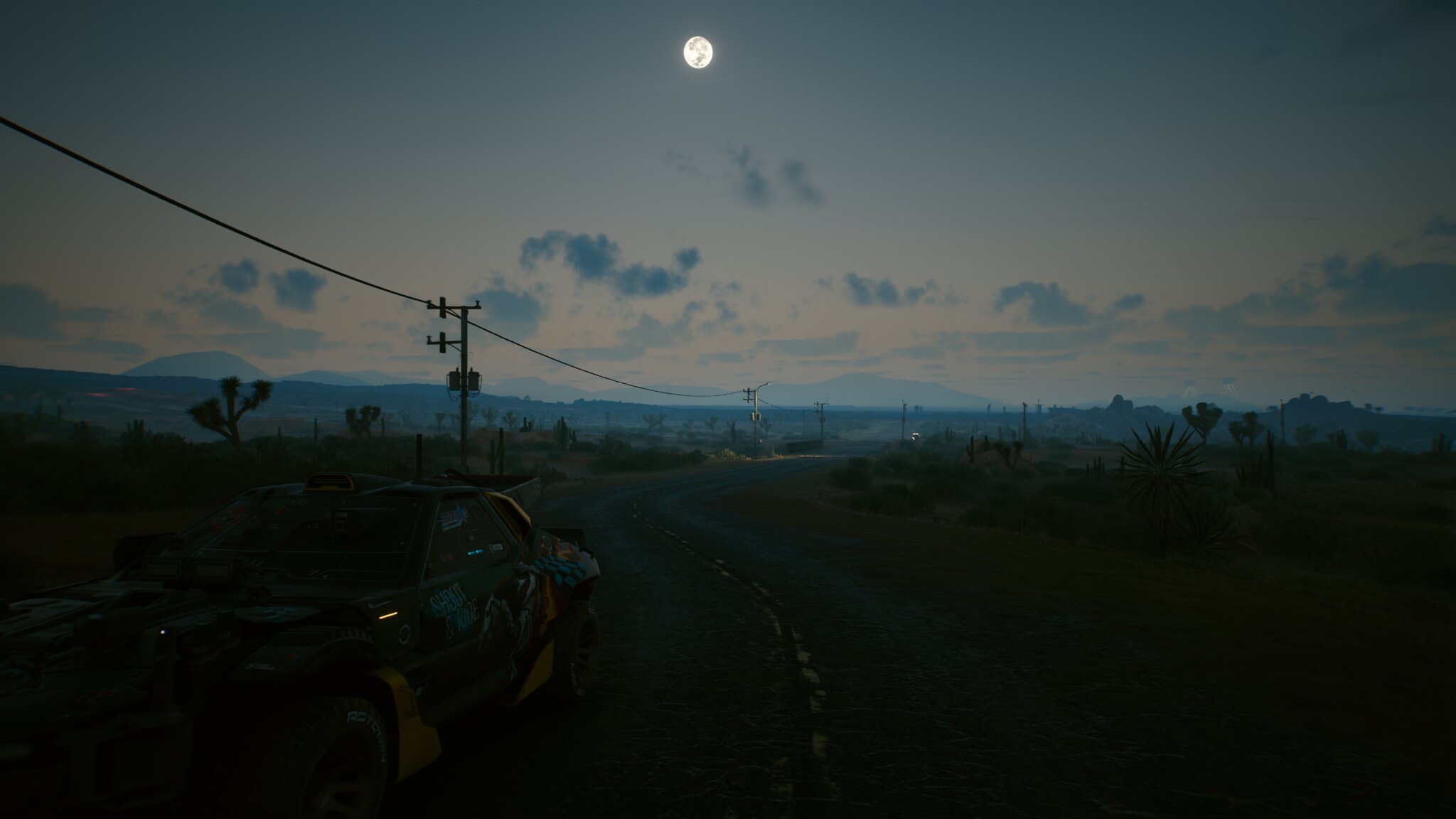In the image, a solitary, sleek black car with yellow accents and black wheels navigates a winding two-lane road through a vast desert landscape. The scene is set around dusk, with the sky painted in deepening hues of twilight, dotted with a few clouds and the faint glow of the moon. Power lines stretch across the open expanse, which is sparsely populated with cacti and other desert vegetation, reminiscent of a setting in Nevada. The car, which resembles a drag racing vehicle equipped with notable side features and possibly extra lights, is the only vehicle on the road, enhancing the sense of isolation and solitude in this serene, almost dark desert environment.